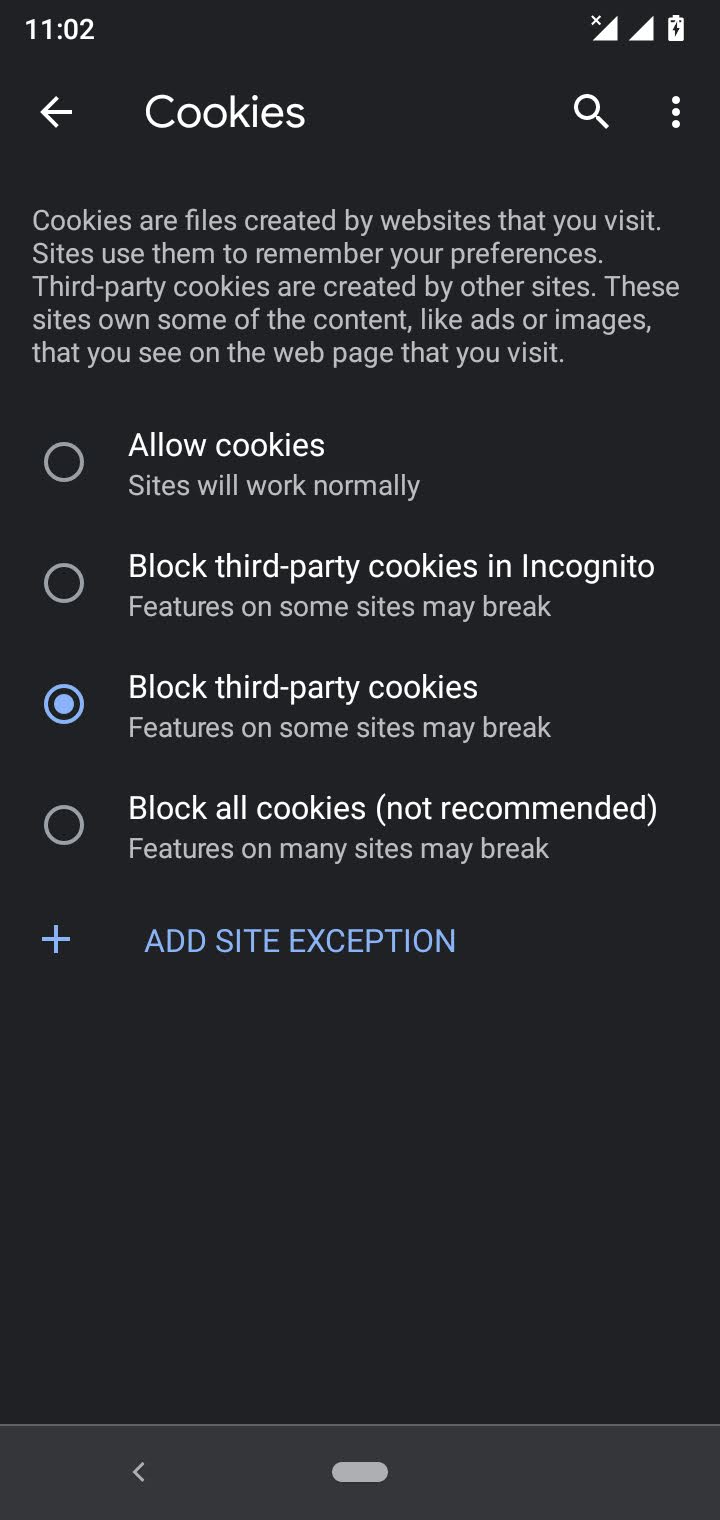A screenshot taken from a cell phone displays a black background with white text. In the upper left corner, the time is noted as 11:02. The upper right corner indicates both a full battery and strong reception. Below these indicators, a search bar contains the word "cookies" with a magnifying glass icon to its right and an arrow to its left.

Following the search bar, an informative text states: "Cookies are files created by websites that you visit. Sites use them to remember your preferences. Third-party cookies are created by other sites. These sites own some of the content, like ads or images, that you see on the web page that you visit."

Underneath this explanation, a list of cookie settings is presented with accompanying round selection circles:
1. **Allow cookies**
2. **Block third-party cookies in incognito**
3. **Block third-party cookies** (with this option highlighted in blue)
4. **Block all cookies** (not recommended)

At the very bottom, in blue text, a plus sign and the phrase "Add site exception" offer an additional option.